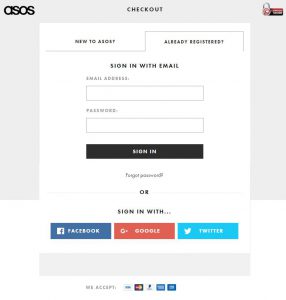The image features a light gray border at the top left and right. In the top left corner, "ASOS" is written in bold black lowercase letters, followed by "CHECKOUT" in small black capital letters to the right. Adjacent to this, there is an icon of a lock accompanied by a red and black box with some text next to it.

Beneath this header, there is a white box. In the top left of this box, it says "New to ASOS?" and to the right, it says "Already registered?". Below, in bold black capital letters, is the text "SIGN IN WITH EMAIL". Beneath this, in gray letters, it says "Email address" with a text box provided below it. Further down, "Password" is written with another text box below it. Underneath these text boxes, there is a black rectangle button that says "SIGN IN". 

Below the button, the text "Forgot password?" is displayed. Further down, there is a line of text that says "OR SIGN IN WITH" followed by icons for various social media platforms: a blue Facebook icon, a red Google icon, and a blue Twitter icon on the right.